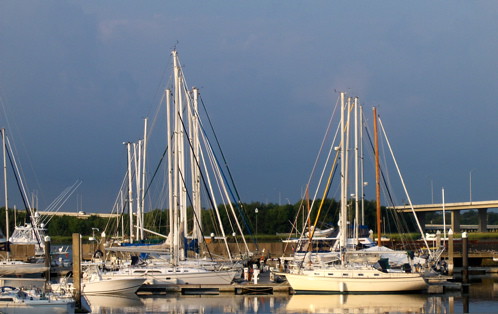This photograph, wider than it is tall, captures a scene at a marina featuring at least four white boats or yachts, arranged in rows. These vessels, with their tall masts, stand against a backdrop of a blue but slightly gloomy sky, hinting at rain. The horizon is lined with green trees, and in the distance to the right, you can see part of a freeway bridge with metal posts extending up from the ground. The reflection of the boats is visible in the water, adding to the serene atmosphere. One of the boats has a distinctive brown mast among the predominantly white ones. The image, though somewhat low quality, provides a detailed view of the marina's boats and surrounding landscape.